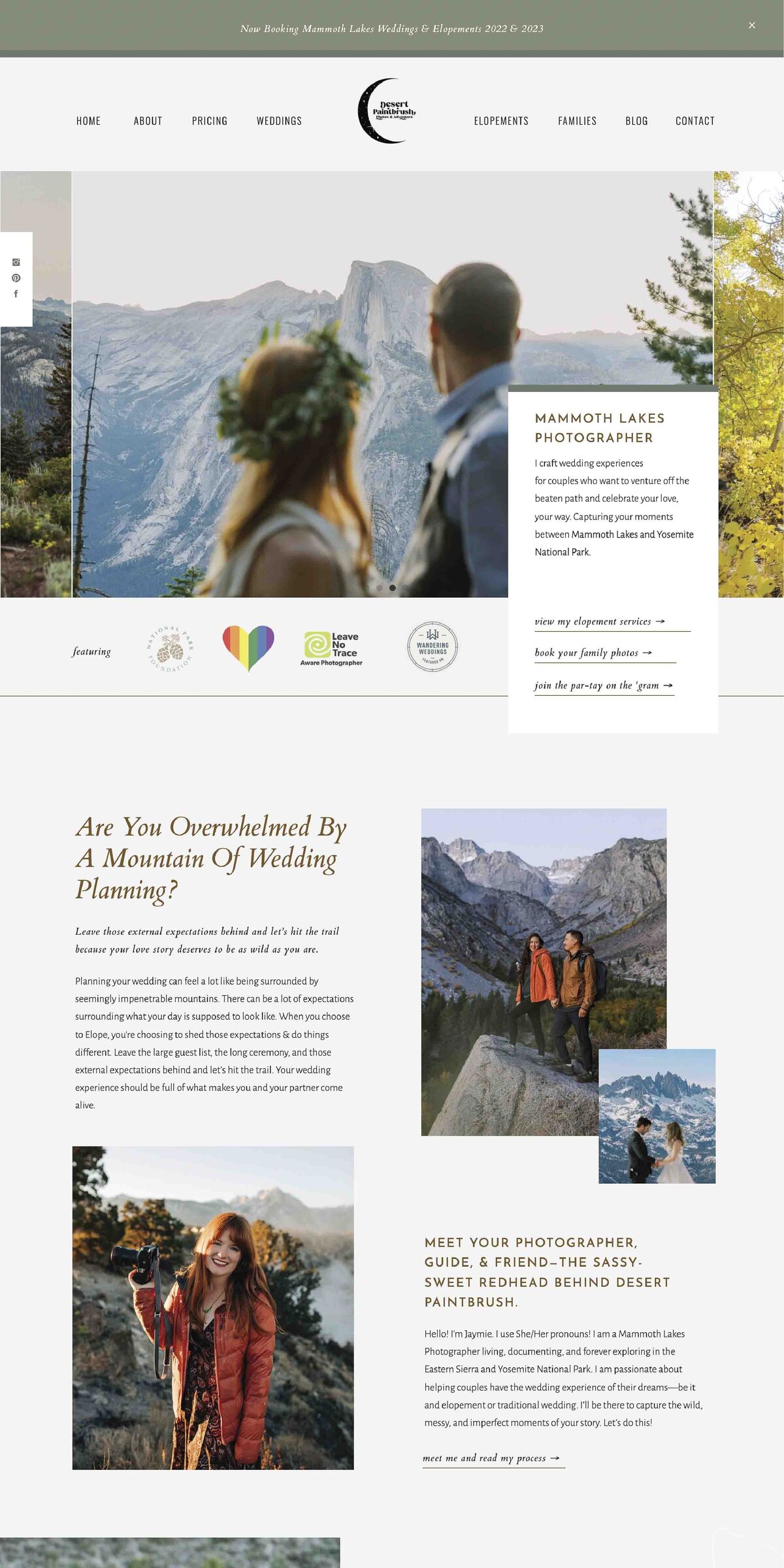This captivating image by Desert Paintbrush perfectly captures the essence of adventure and romance. At the top of the page, there's a navigation menu offering options for Home, Pricing, Weddings, Elopements, Families, Blog, and Contact.

The photograph features a Caucasian couple centered within a larger white background, almost as if it’s a picture within a picture. The bride, with her flowing reddish-brown hair adorned by a delicate green wreath, is dressed in a sleeveless top. Beside her, the groom, seen in a side profile, wears a collared shirt with a low haircut, coupled with a long blue-sleeve shirt. They both gaze towards a majestic mountain range, partially covered in snow, with lush green trees dotting the landscape.

A message overlay introduces the photographer, stating, "I craft wedding experiences for couples who want to venture off the beaten path and celebrate your love your way." She offers an array of services including elopements, family photos, and invites visitors to join the community on Instagram. She proudly showcases her affiliations with the National Park Foundation, highlights her support for the LGBTQ community with a rainbow heart, and promotes being a Leave No Trace Aware Photographer and a member of Wandering Weddings.

An inspiring call to action reads, "Are you overwhelmed by a mountain of wedding planning? Leave those external expectations behind and let's hit the trail because your love story deserves to be as wild as you are." Underneath this, various images depict couples engaging in non-traditional wedding settings; one couple hikes in casual attire with jackets and backpacks, while another embraces in wedding attire on a mountainside.

Lastly, meet Jamie, the sassy and sweet redheaded photographer behind Desert Paintbrush. She is shown outdoors, camera in hand, donning an orange puff jacket and a brown floral skirt, embodying the adventurous spirit she brings to her work.